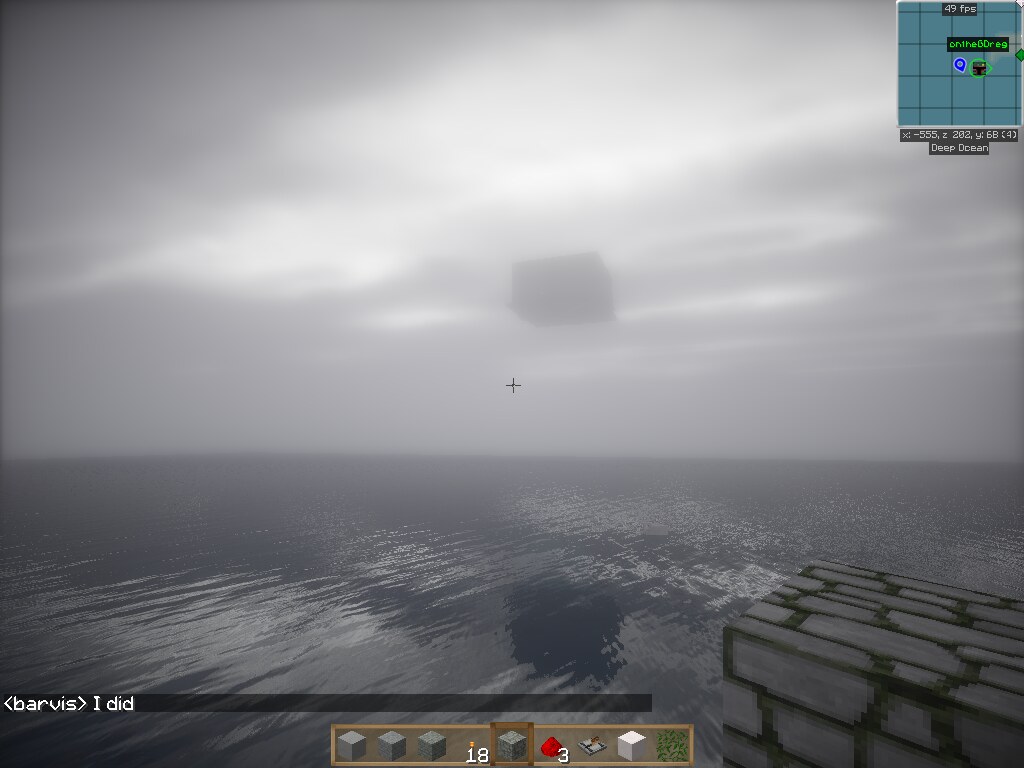This still image from a Minecraft video game features a serene open water scene beneath a vast expanse of sky. Occupying the upper two-thirds of the frame, the sky is predominantly gray, interspersed with sparse, hazy white clouds that appear spread out rather than fluffy. In the upper right corner of the image, a blue-gray square grid is visible, indicating performance statistics with "49 TPS" displayed prominently in white text on a black rectangle at the top center. Below this, it reads "online 6th" with a series of icons and notations indicating player positioning. Further text with numerical data appears beneath, along with the label "deep ocean." A faint rectangular shadow can be seen in the background sky, adding an element of intrigue to the scene. The image captures a moment of tranquility in the game, inviting viewers to appreciate the virtual seascape and sky.